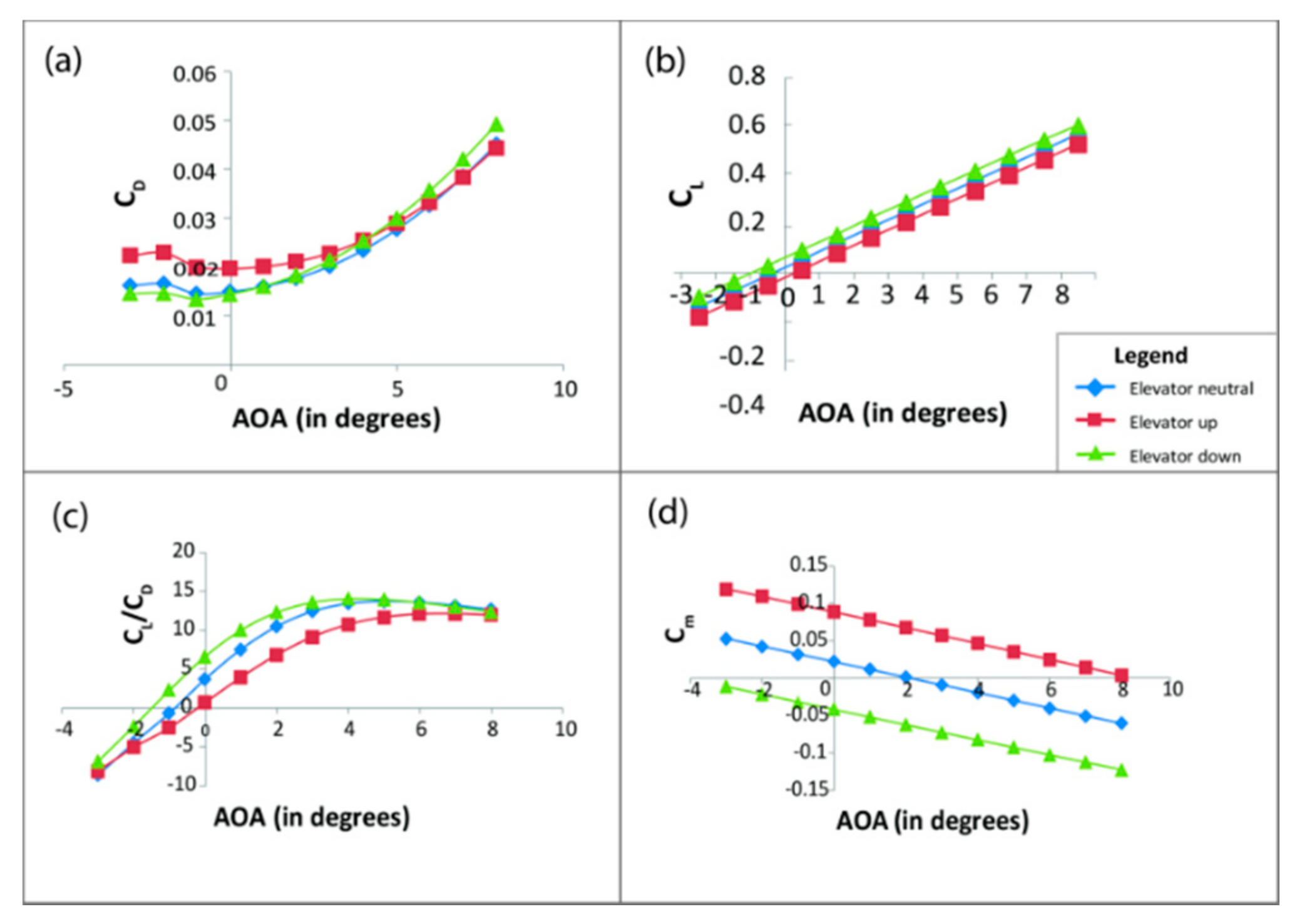The image shows four distinct rectangular charts arranged in a 2x2 grid, each labeled in the upper corner with alphabetic identifiers A, B, C, and D. All charts display data along an x-axis labeled "AOA in degrees," ranging from 0 to 10 degrees. Each chart also has a different y-axis, with units like degree centigrade, CL/degree centigrade, and other variables denoted by C with subscripts such as L and E.

Each chart features three data lines distinguished by color and shape: a green line with triangles, a blue line with squares, and a red line with squares. The legend, positioned within one of the charts, clarifies the data representations: the blue line with squares indicates "elevator neutral," the red line with squares denotes "elevator up," and the green line with triangles represents "elevator down." These line graphs plot approximately 12 data points across the specified range on the x-axis, providing multi-faceted insights into the variables measured on the y-axes.